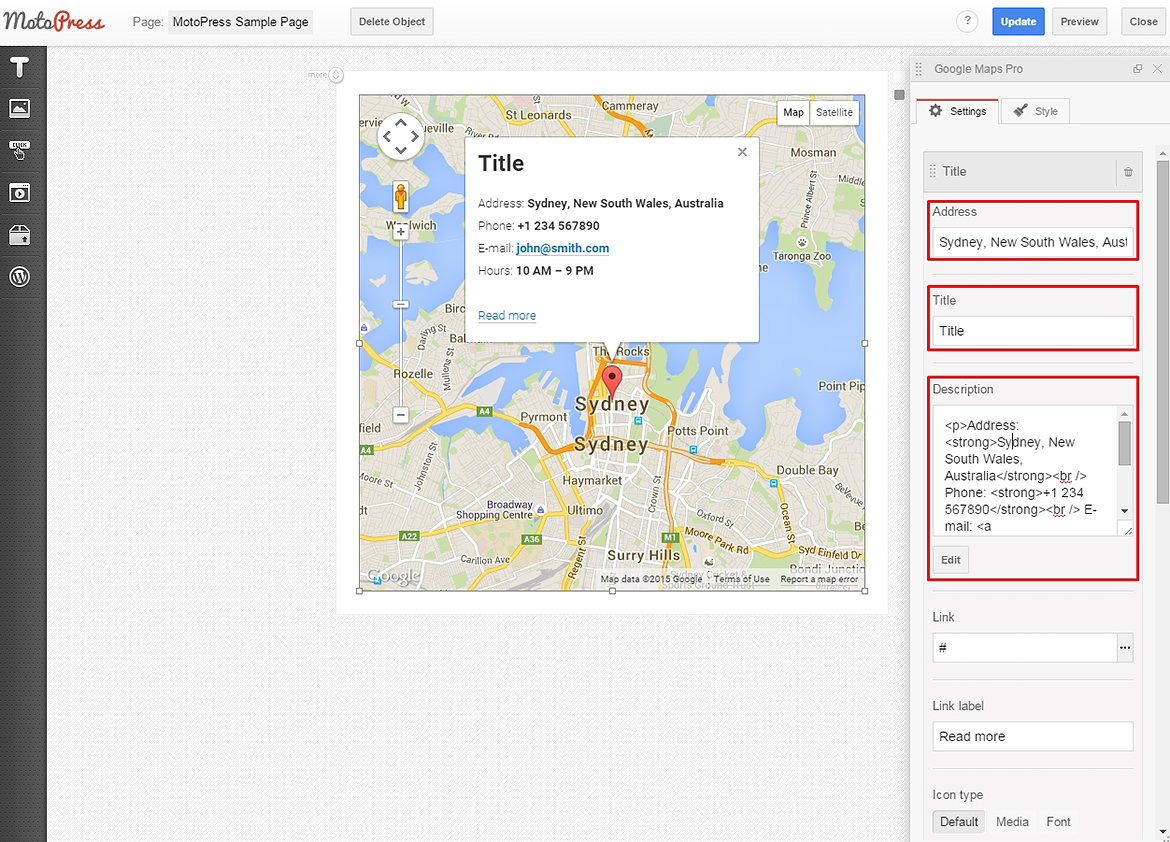The screenshot showcases the interface of Modo Press, highlighting various elements and settings options for editing a page titled "Sample Page". The primary focus is on several action buttons and input fields.

### Main Interface Elements:
- **Buttons:**
  - **Update:** Featured in a blue rectangle, indicating its prominence.
  - **Preview, Close:** Additional options presented within rectangular buttons.
  - **Delete Object, Question Mark:** Likely tools for modifying or seeking help.

### Content Blocks:
- **Title and Contact Information:**
  - **Title Field:** Contains the heading for the section.
  - **Address Details:** Provides specific contact information, including:
    - **Location:** Sydney, New South Wales, Australia.
    - **Phone:** +1-234-567-890.
    - **Email:** john@smith.com (hyperlinked for direct email setup).
    - **Operating Hours:** 10 a.m. to 9 p.m.
    - **Read More:** A hyperlink leading to additional information.

### Map Display:
- **Visuals:** Features a map with an overlaid square containing the above-mentioned contact information.

### Sidebar Options:
- **Settings Panel:**
  - **Sections:** Include Title, Address, with fields repeating the same contact information.
  - **Google Maps Pro Settings:**
    - **Styles and Settings:** Multiple tabs available with the "Settings" tab currently selected, indicated by a red line.
  - **Fields:** Include Title, Description, and some coding snippets such as P and Address tags.

This detailed caption describes the screenshot comprehensively, capturing all elements and their layout within the Modo Press interface.